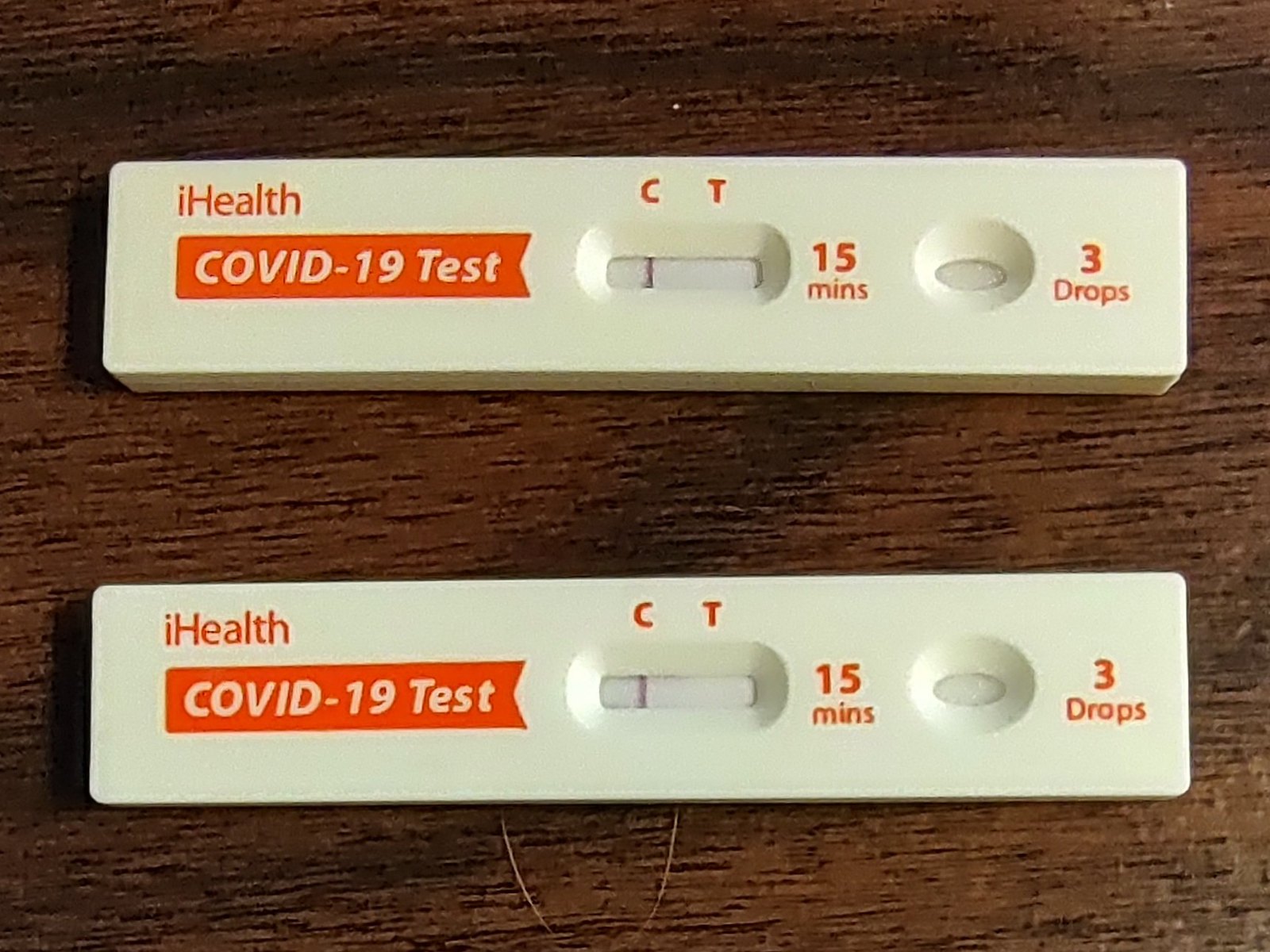The image depicts a wooden brown surface with two iHealth COVID-19 test strips placed on top. The test strips are identical, labeled with orange ink, and indicate that the test duration is 15 minutes, requiring three drops to function. Both test strips appear to have been used. Each strip has the letters "C" and "T" marked, with a white background resembling a small screen. A single red line is visible next to the "C" on both strips, suggesting a negative result for the iHealth COVID-19 test.